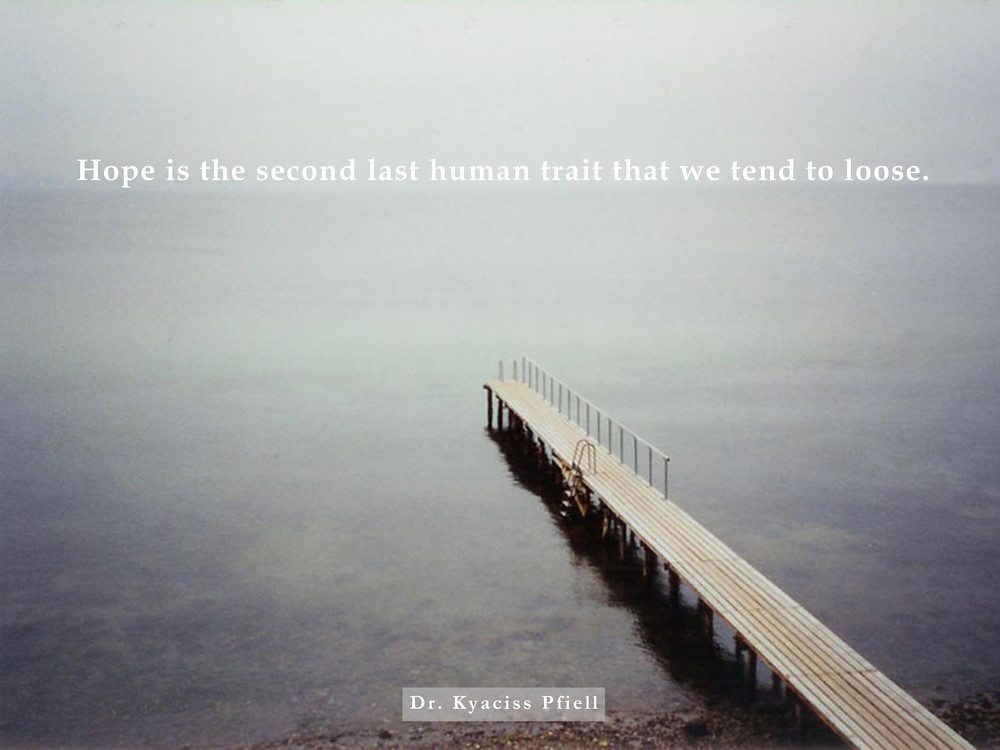This image shows a tranquil, misty scene featuring a narrow, wooden pier extending into still, gray water, with a single metal railing on the right side and a small ladder leading down. Both the water and sky merge into an almost indistinguishable gray horizon, creating a serene yet somber atmosphere. At the top of the image, the phrase "Hope is the second last human trait that we tend to lose" is prominently displayed in white text, slightly misspelled as "L-O-O-S-E." At the bottom, the name "Dr. Kaya's File" is centered in white text, suggesting that this may be an inspirational or motivational graphic, possibly of a religious nature, though the exact context is ambiguous.